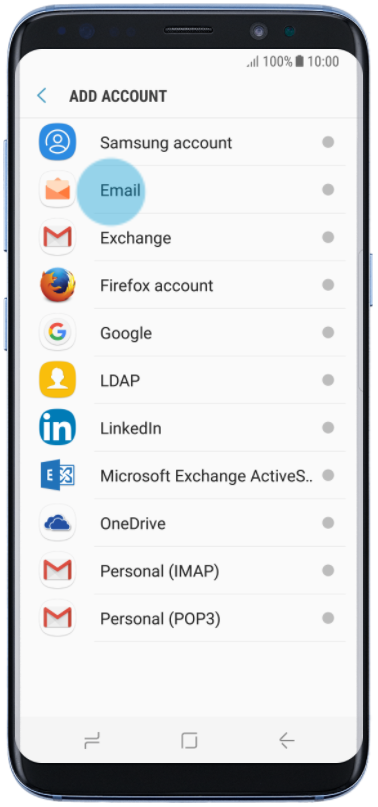A detailed photo of a smartphone screen displaying various account options and their respective icons. The image features the following elements:

- **Phone Frame and Status Bar**: The phone's black outline surrounds a white screen. In the upper right-hand corner, icons indicate full phone signal strength (displayed as black bars resembling a staircase) and battery status at 100% with a black percentage symbol and a fully charged battery icon. Below these icons, text reads "10:00".
  
- **Add Account Section**: On the left side of the screen is a blue arrow pointing to the left, followed by the text "Add account" in black. 

- **Account List**:
  - **Samsung Account**: Next to a blue box featuring a white outline of a person, it says "Samsung account" in black text, accompanied by a gray circle to the right.
  - **Email**: Represented by a white box with a green envelope icon containing a lighter green piece of paper. The black text "Email" is circled by a blue ring, with a small gray circle to the right.
  - **Exchange**: Indicated by a white circle with a red "M" inside. The word "Exchange" appears in black text, flanked by a gray circle.
  - **Firefox Account**: The Firefox logo (a blue sphere with a reddish-yellow fox curled around its bottom) is shown with the black text "Firefox account" nearby.
  - **Google**: A white circle with the multicolored Google logo (red, yellow, green, and blue) inside a red box. The text "Google" appears in black.
  - **LBAP**: Represented by a yellow box containing a white silhouette of a person's head. The letters "LBAP" appear in black text.
  - **LinkedIn**: Shown as a blue box with "IN" in white letters, followed by the black text "LinkedIn".
  - **Microsoft Exchange Activity**: A blue piece of paper with a white "E" and a blue page outline featuring butterfly wings. The gray text reads "Microsoft Exchange Activity S…" (trailing off).
  - **OneDrive**: Two blue cloud icons in a white box, accompanied by the text "OneDrive" in black.
  - **Personal (IMAP)**: A white box with a red "M" and the black text "personal (IMAP)".
  - **Personal (POP3)**: Another white box with a red "M" next to the text "personal (POP3)" in black.

Each account entry has a corresponding gray circle on the right-hand side, visually aligning the options in a structured layout.